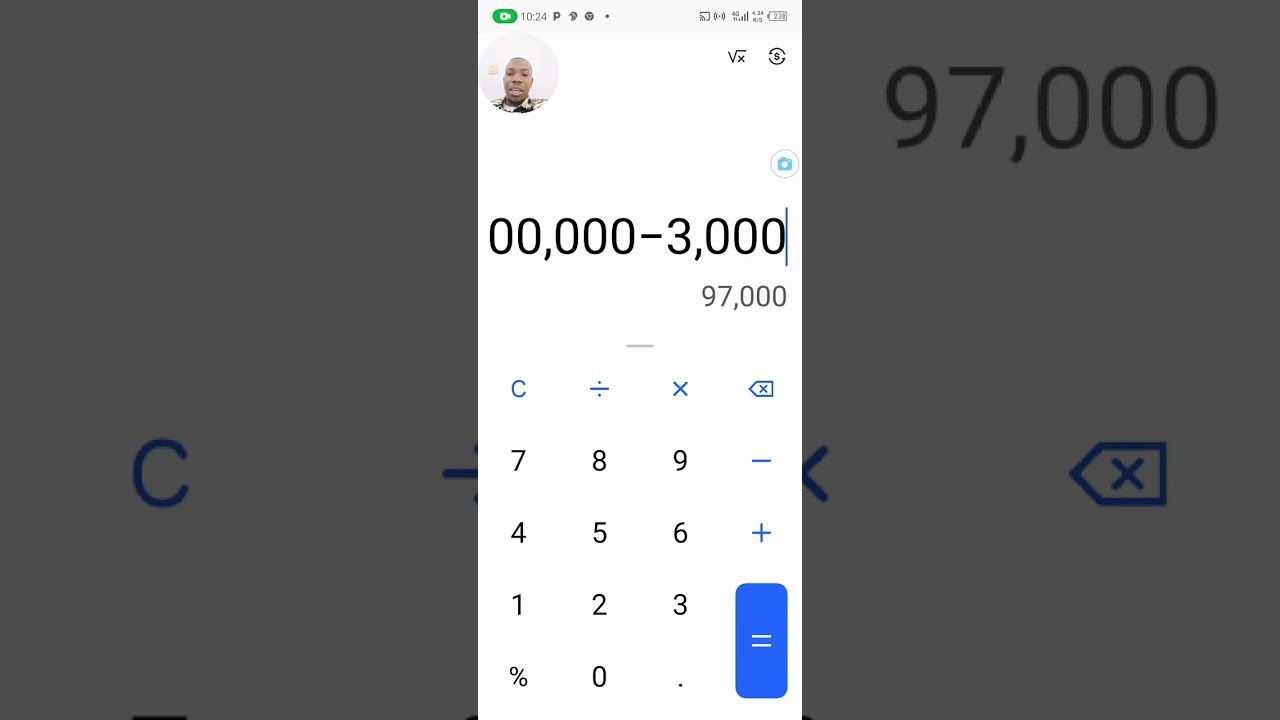This image is a detailed screenshot of a calculator app on a smartphone, featuring a diverse range of icons and functions. The display is divided into three main sections. At the very top, the screen shows typical smartphone icons: on the left, the time reads 10:24, accompanied by an icon of a smiling black man in a small circle, hinted to be the owner of the phone or perhaps instructing on its use. The upper right corner displays the battery indicator, signal strength, and Wi-Fi icons. 

The middle section is dominated by the calculator app on a white background. At the center, the calculation "100,000 - 3,000" is prominently displayed, with the result "97,000" shown below it. A sequence of calculator buttons follows, including a blue bar with the symbols: C (clear), division (÷), multiplication (×), and a delete key (del). This is trailed by the numeric pad in a standard layout (7, 8, 9, -, 4, 5, 6, +, 1, 2, 3, =, 0, .), all set in black font with a blue equal sign button. 

Among these buttons, special symbols are noted: a percent sign (%) in the bottom left corner and a zero (0) encircled in gray. Additionally, there are some function icons: a square root with an X, an S with a circle around it, a line with arrows pointing left, and another with circles pointing right. Flanking the calculator display are close-ups: on the left, the seek button, and on the right, the delete key.

The overall image captures a comprehensive and instructive view of using the calculator app on a smartphone, possibly being demonstrated by the individual whose profile appears in the upper left.